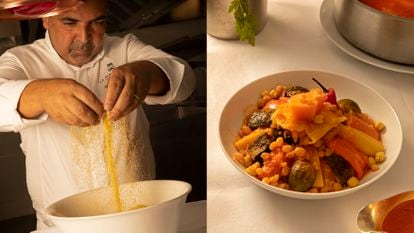The image features two frames placed side by side. In the left frame, there's a chef dressed in a white chef's outfit with folded sleeves. He is actively preparing a meal, mixing ingredients with his hands in a white bowl that contains yellow and grain-like items. In the right frame, the finished dish is presented—a vegetarian pasta dish in a white ceramic bowl. The dish includes beans, pasta, carrots, small red peppers, and possibly corn. The bowl sits on a white table, surrounded by additional plates and sauce bowls, with a pot visible in the top right corner. The setting is well-lit, providing a clear view of both the preparation process and the final presentation.